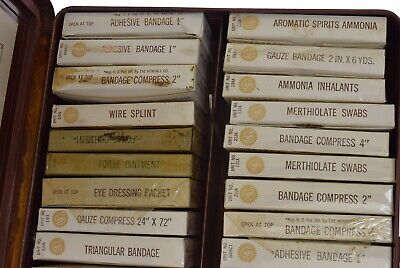The image portrays the contents of an old first aid kit neatly organized in a rusty, brown container that resembles a cassette tape case. Inside, the faded white boxes, each roughly the size of a cassette tape and featuring yellow circles on the left edge, are meticulously arranged in two tight columns of about nine or ten boxes each, with a slight gap between the columns. The spines of the packages, labeled in red text, face upwards and include various medical supplies such as adhesive bandages, triangular bandages, compressed gauze, wire splints, aromatic spritz ammonia, ammonia inhalants, methiolate swabs, and bandage compresses of various sizes. The labels and the aged appearance of the boxes suggest that this first aid kit dates back to the 1960s, 70s, or 80s.